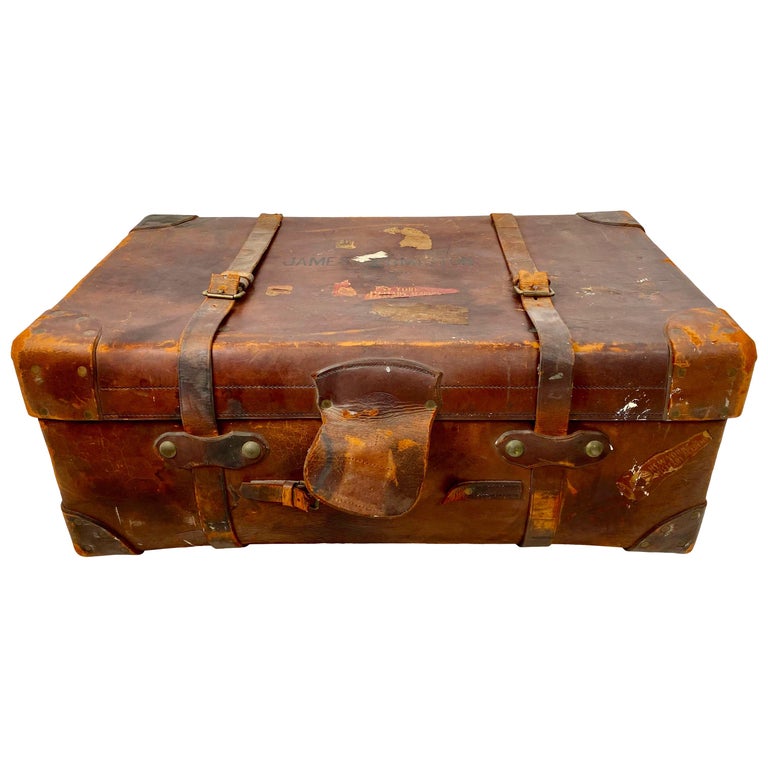This detailed image showcases a very old, brown leather traveler's trunk, appearing vintage, potentially over 100 years old. The suitcase exhibits significant wear and tear, with lighter orange patches and edges where the leather has worn away, revealing a distressed, well-traveled look. Silver bolts and metal ends secure the corners of the trunk, adding a touch of durability to its aged aesthetic. Leather straps encircle the suitcase, but their exact fastening mechanism remains hidden. A flap of leather covers what might be a lock or a closure system, adding to the mystery of its function. There's some faint printing on the top, partially legible to spell out "James," but the rest of the text is unreadable. The suitcase is set against a pristine white background, ensuring that its vintage charm is the focal point.